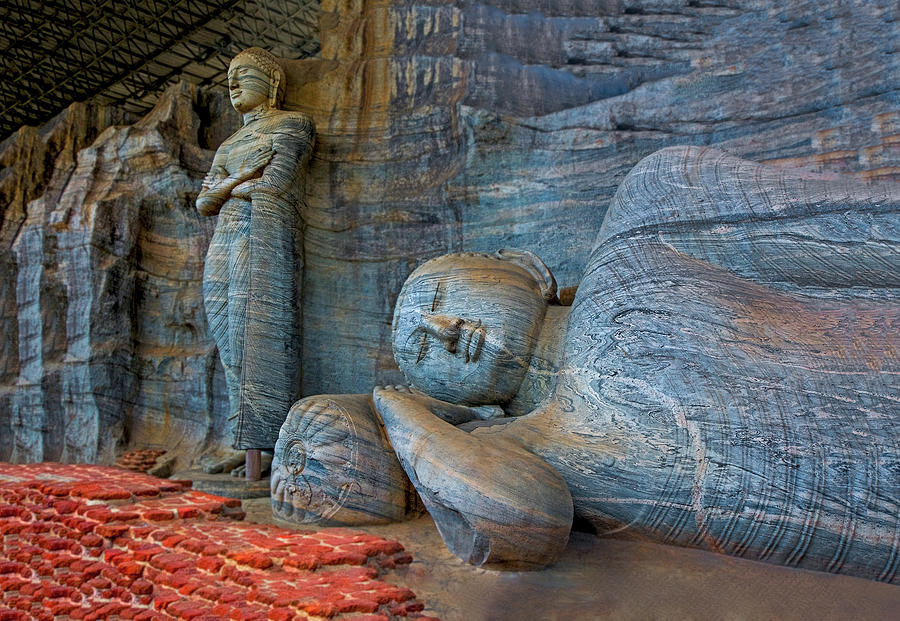This image depicts a detailed stone carving inside what appears to be a cave or Buddhist temple, showcasing two Buddha statues. The first Buddha stands upright with arms crossed over the chest, exuding a traditional, serene expression with finely chiseled facial features. The second Buddha, positioned to the side, is reclining with a small cylindrical pillow adorned with a flower under its head; only its upper body, including the head and torso, is visible. The statues are carved from a rock face with a distinct bluish-gray hue and intricate detailing, reflecting exceptional craftsmanship. The scene is framed by a large metal overhead structure, and the floor in front of the statues is strewn with red objects resembling stones or possibly raw meat, adding a stark contrast to the grayscale surroundings. The entire tableau captures the essence of ancient Asian art, with meticulous attention to the facial features and drapery of the figures.